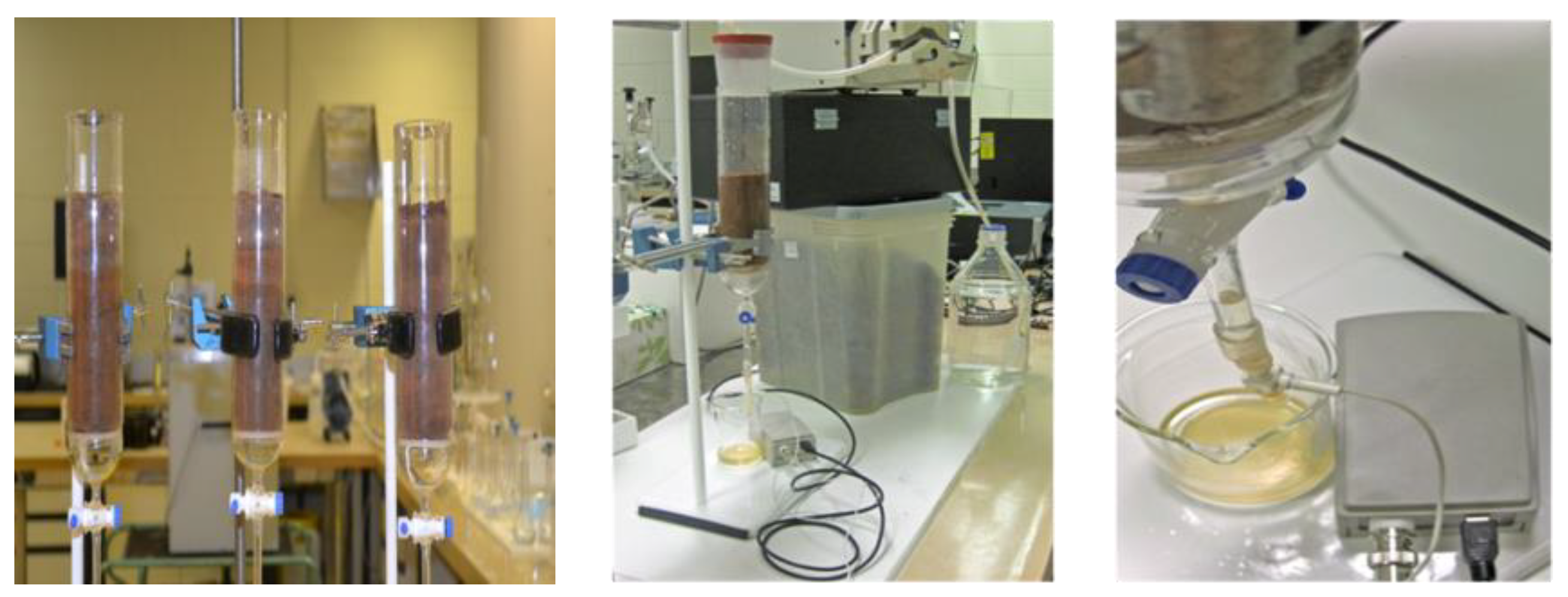A horizontally arranged triptych features detailed images of laboratory equipment, each divided by a white bar. The leftmost photo displays three transparent cylinders, each about 75-80% filled with a light pinkish liquid, with tubes extending from their bottoms. Behind these cylinders, a countertop is visible, cluttered with an assortment of additional glassware. The central image highlights a container topped with a black box, surrounded by various electronics and wires. Tubes loop into clear bottles filled with differing liquids, adding to the scientific intricacy. The rightmost photograph offers a close-up of a glass measuring cup being filled from a clear tank above it. This setup, entwined with tubes, also features a gray box equipped with connectors. The entire composition is set against a stark white background, emphasizing the precision and cleanliness of the laboratory environment.